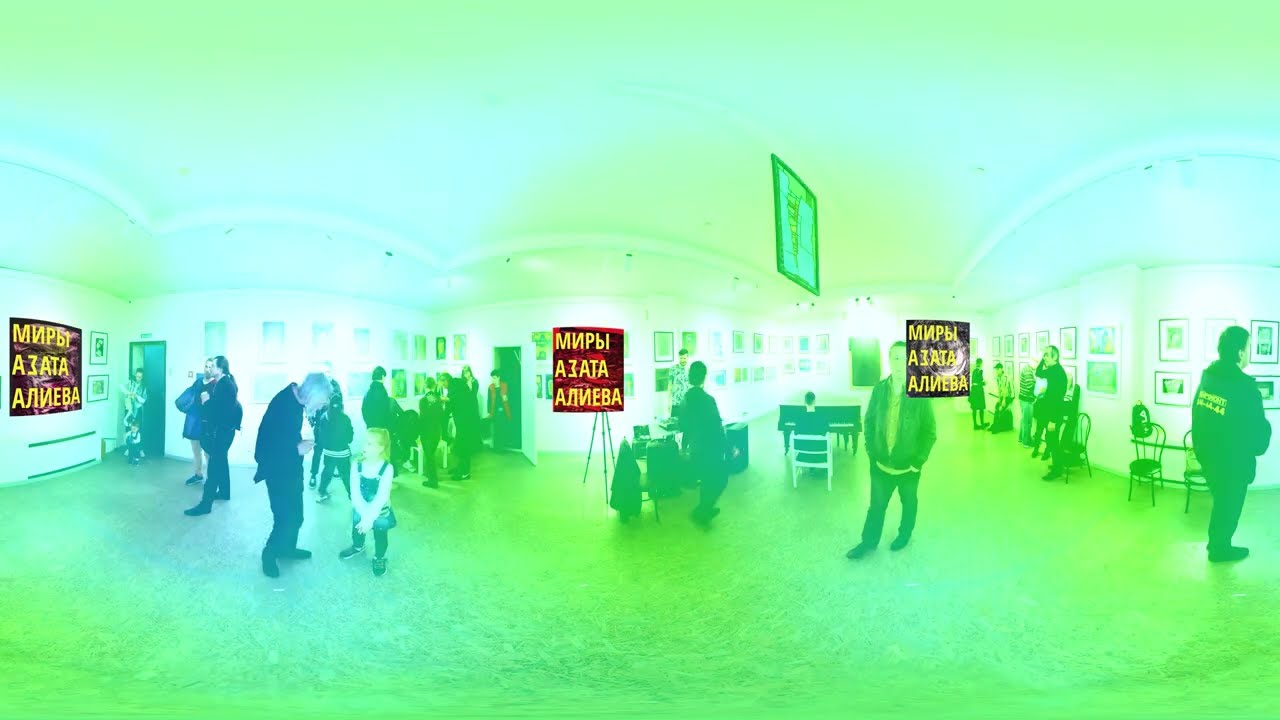The image depicts the interior of a museum or an office lobby, captured with a wide-angle lens. The scene is modified with a surreal green and blue aurora-like filter, giving the image an otherworldly glow. The room is bathed in light with walls adorned with multiple rows of square-framed portraits and photographs. People are scattered throughout the space: some are gazing at the artwork, others are mingling or walking about. Notable interactions include a man conversing with a young girl in overalls, and another man wearing a suit talking to someone with a bag. A woman is seen entering through a door. Adding to the surreal quality, there are three superimposed square overlays with purple and red backgrounds featuring yellow writing in an undecipherable foreign language. These overlays appear to be digitally added, partially covering some of the figures in the image. The roof, mostly white but also tinted green, has banners hanging that display an indiscernible sequence of letters. Overall, the scene combines the everyday tranquility of a museum visit with fantastical and digital elements.